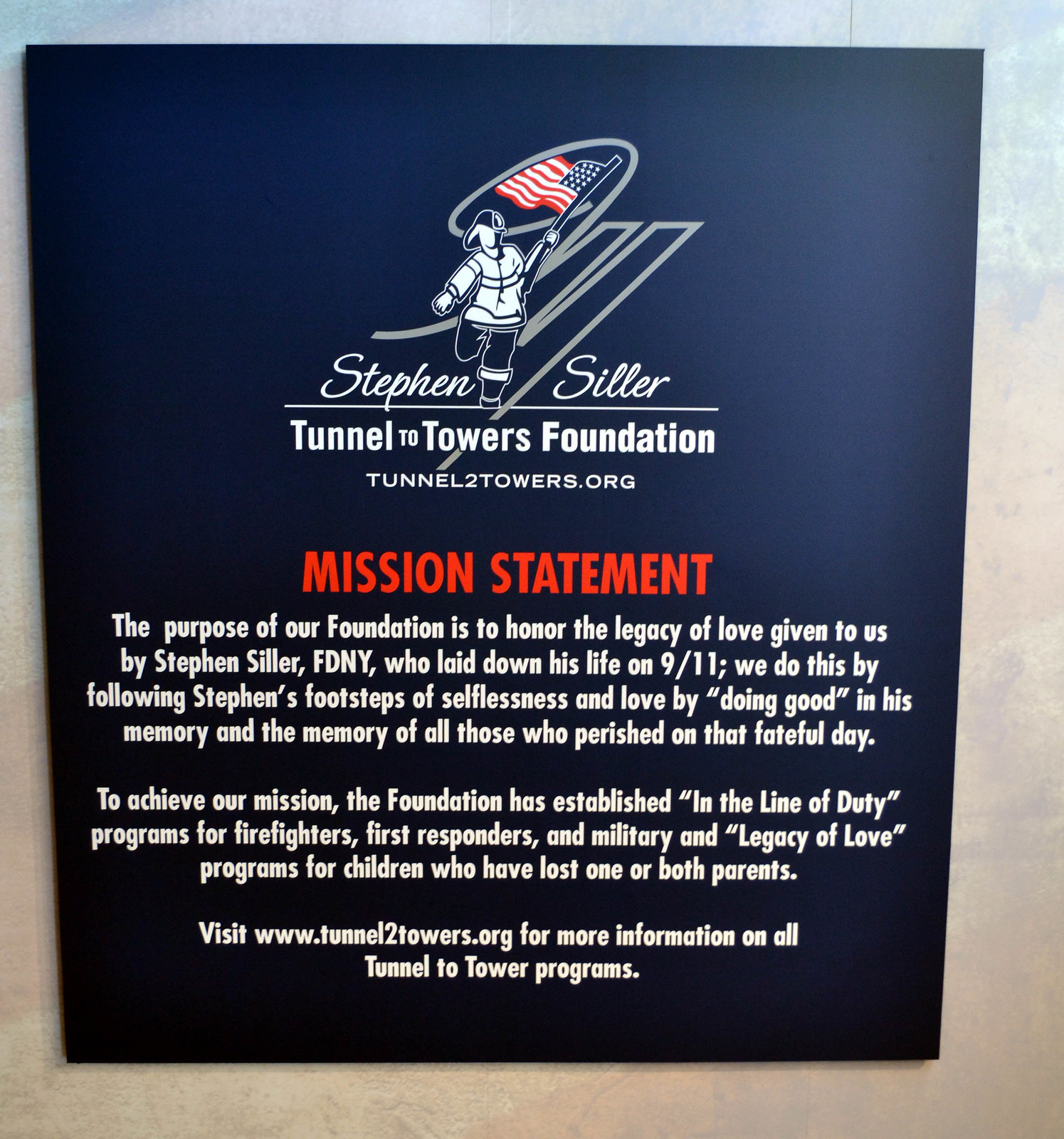The image depicts a vertical, navy blue poster affixed to a light gray wall with a touch of light blue at the top. Dominating the poster is a cartoon illustration of a firefighter in a baseball uniform running towards the viewer while holding an American flag in the left hand. Above this illustration, in bold white text, is the heading "Stephen Siller Tunnel to Towers Foundation" followed by the organization's website, "TunnelTwoTowers.org." Below this, in capitalized red letters, is the title "Mission Statement." 

The mission statement is detailed in white text, occupying the lower half of the poster. It reads: "The purpose of our foundation is to honor the legacy of love given to us by Stephen Siller, FDNY, who laid down his life on 9/11. We do this by following Stephen's footsteps of selflessness and love by doing good in his memory and the memory of all those who perished on that fateful day. To achieve our mission, the foundation has established in-the-line-of-duty programs for firefighters, first responders, and military, and legacy of love programs for children who have lost one or both parents. Visit www.tunneltotowers.org for more information on all Tunnel to Towers programs."